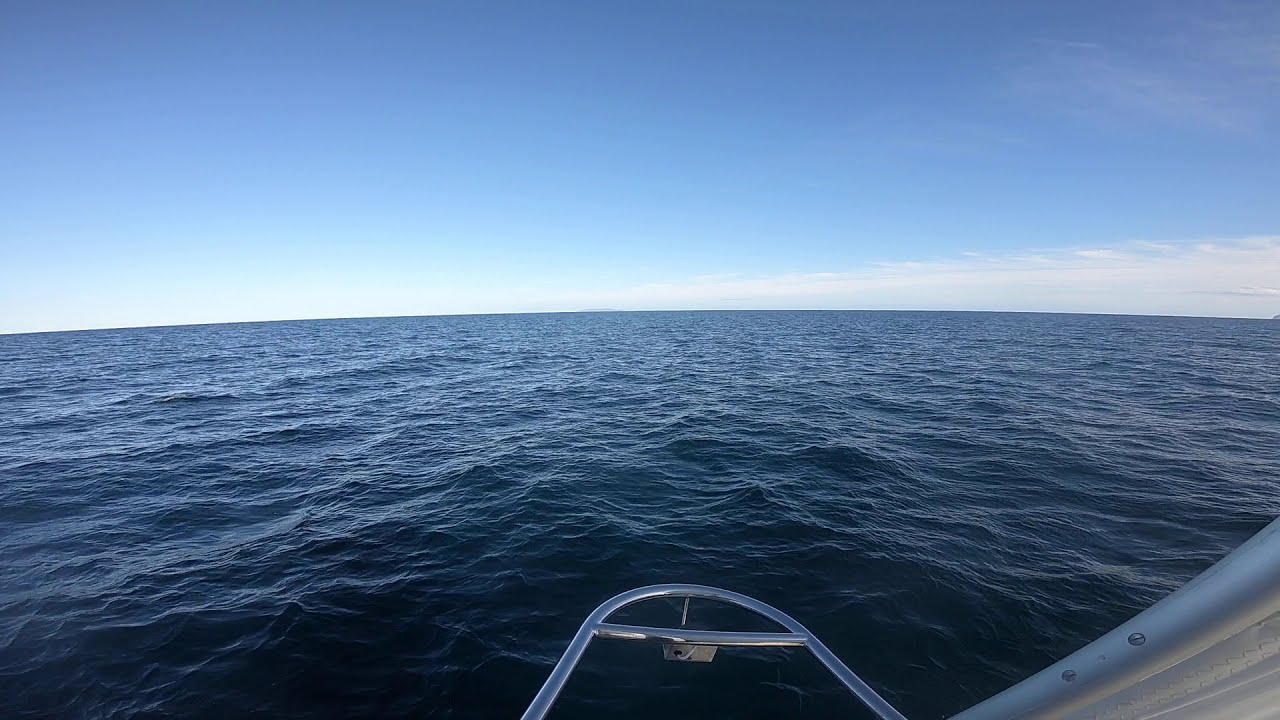This is a detailed exterior daylight photograph of the open ocean, taken from the front of a boat. The scene is dominated by choppy, dark blue waves that extend from the foreground to the distant horizon. The surface of the water is rougher near the boat and smooths out as it recedes into the distance. The sky above is a serene light blue, mostly clear but dotted with a few wispy white clouds concentrated toward the upper right part of the image. In the bottom right of the photograph, part of a boat is visible: a silver structure with metal tubes forming a reverse U-shape, likely part of a railing or an anchor system. This metallic assemblage suggests the viewpoint is from the boat itself. To the far right on the horizon, a small portion of land is faintly visible. The overall composition captures the vastness and tranquility of the sea on a clear day, emphasizing the seamless transition between the deep blue waves and the pale blue sky.